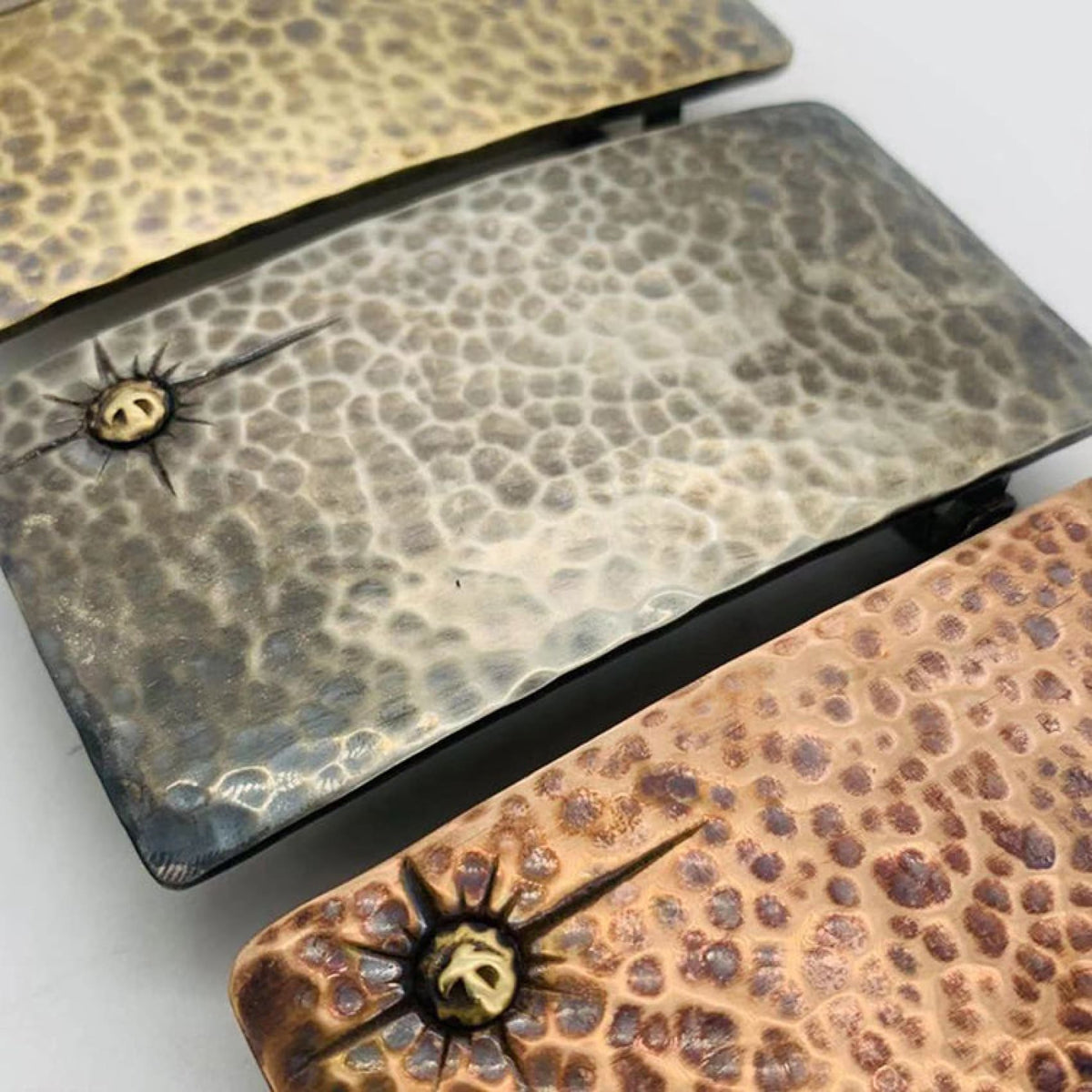The photograph showcases three textured metal belt buckles arranged on a smooth, light gray surface, likely a table or counter. Each buckle mimics the appearance of lizard skin through a hammered and burnt metal design. The center buckle is fully visible, displaying a gray hue with dark gray pits. It features a distinct business logo—a gold smiling face set against a black star—in its top left corner. The top left buckle, partially in frame, has a golden color with dark brown pits, and the bottom right buckle, also partially visible, is predominantly brass with dark indentations. All three buckles share the same unique logo and overall design aesthetic.